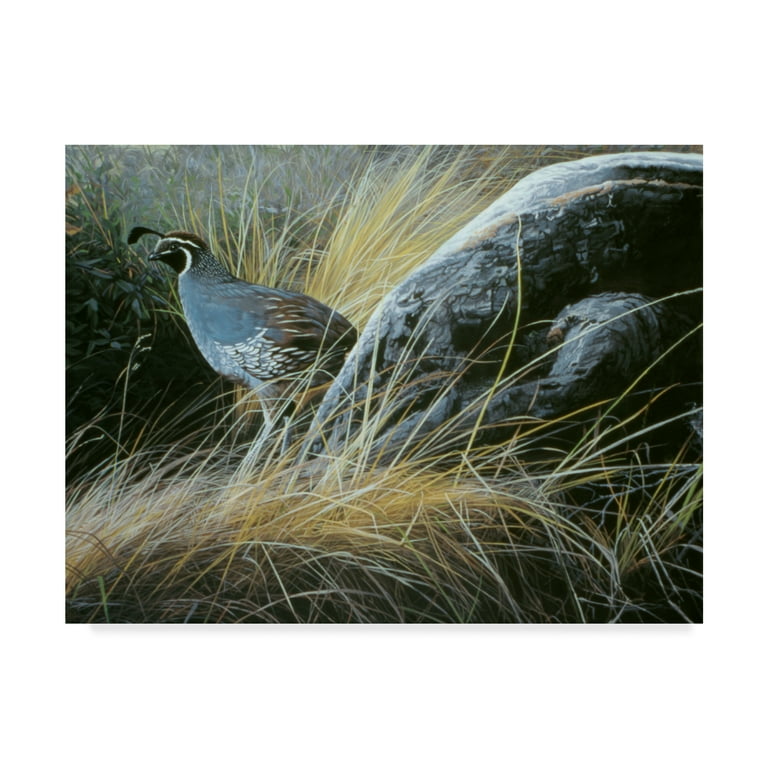The image captures a striking nature scene that appears almost like an oil painting. Dominating the left third of the composition is a bird reminiscent of a peacock or quail, standing in a brushland area. This avian subject boasts a blue body with a white underbelly, brownish feathers on its back, and a black and white head adorned with a distinctive tuft of feathers that protrudes like a unicorn horn. The bird's yellow eyes and small black beak are clearly visible as it gazes to the left. The setting features a large, gray rock marbled with white splotches and hints of moss, occupying the majority of the right side of the image. Surrounding this rock and the bird is a sea of tall, overgrown grasses—predominantly brown and yellow—with tinges of green that are too dark to discern clearly. The scene is bathed in the soft light of daytime transitioning into evening, providing a serene yet dynamic backdrop to the tranquil subject.